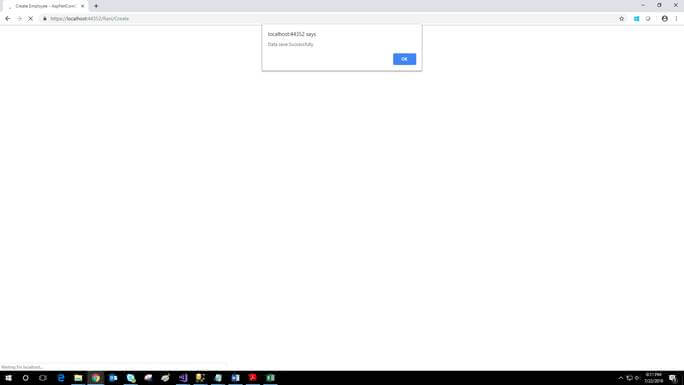The image depicts a Windows Desktop with the taskbar visible at the bottom, featuring various icons. The Google Chrome browser icon is highlighted, confirming that Chrome is the active application. The browser displays a page titled "localhost," followed by a sequence of numbers, indicating a local web server address. 

A dialog box is prominently visible in the center of the screen, stating "localhost says: Data saved successfully," with an "OK" button below it, styled in blue. The main content of the browser page is predominantly empty, showing a blank white space. Additionally, there's a Windows extension icon in the browser, though its function remains unclear due to the low resolution of the image. Some small, indistinguishable text is also present, but the blurriness makes it illegible. Overall, the caption suggests that the operation was successful despite the absence of visible content on the main page.